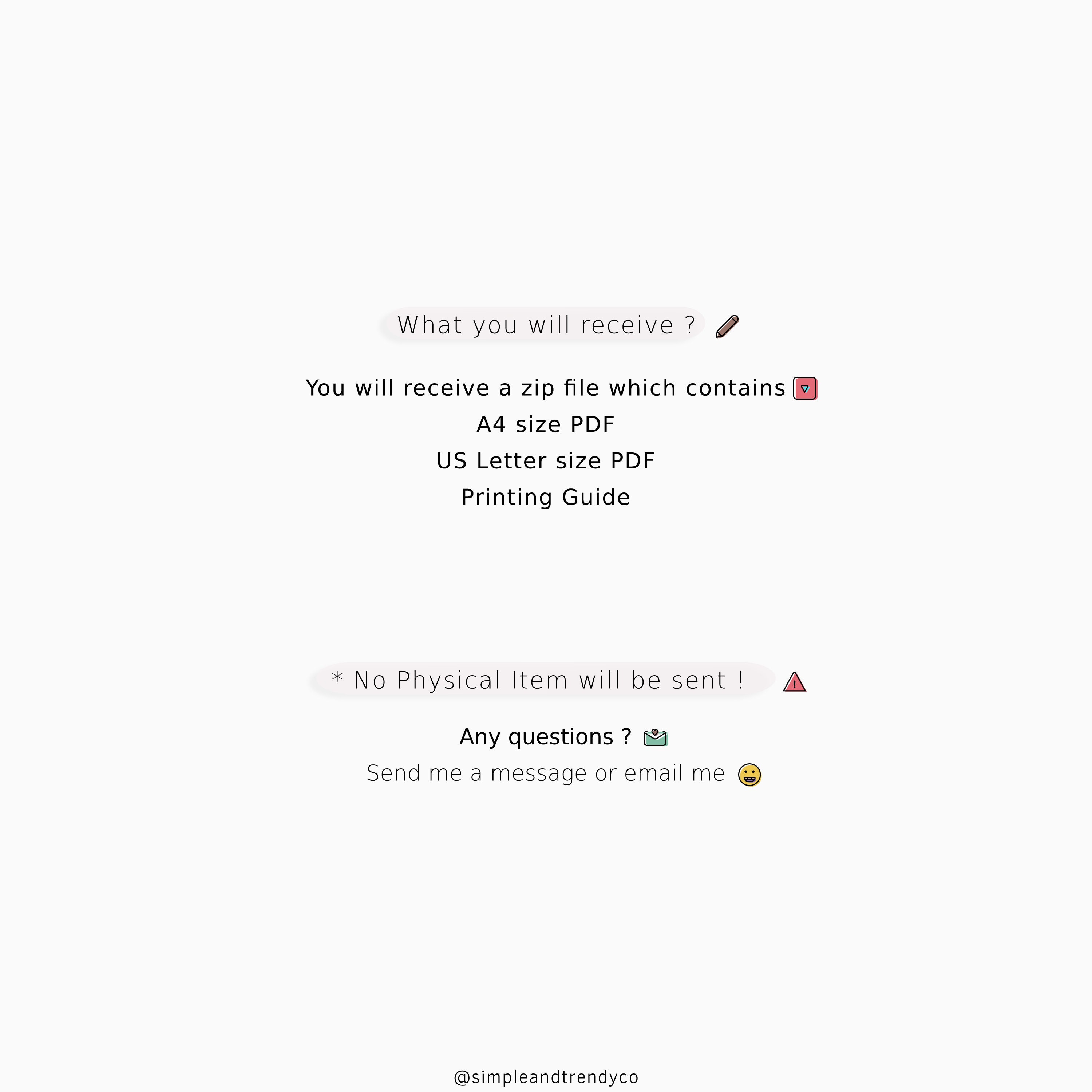**Detailed Caption:**

The screenshot captures a minimalist website layout dominated by white negative space, with all black text centrally aligned. At the top, in very thin black text, the header reads "What will you receive?" accompanied by a small pencil icon to its right. Below this line, bold text states, "You will receive a zip file which contains." To the right of this line is an icon of a black box with a white downward-pointing triangle. 

Following this, the text lists the contents of the zip file in three separate lines:
- "A4 size PDF"
- "US letter size PDF"
- "Printing guide"

After a significant gap of white space, a new header in thin black text declares, "No physical item will be sent!" with a red triangle icon and a black exclamation point to its right. Further down, the bold text "Any questions?" appears, next to a green envelope icon.

Underneath this, in thin black text, it instructs, "Send me a message or email me." Beside this line, there's an icon of an open-mouthed smiley face. Finally, at the bottom of the image, after another large expanse of negative space, the text "@simpleandtrendyCo" appears in small black letters, making it clear that it is styled as a single word.